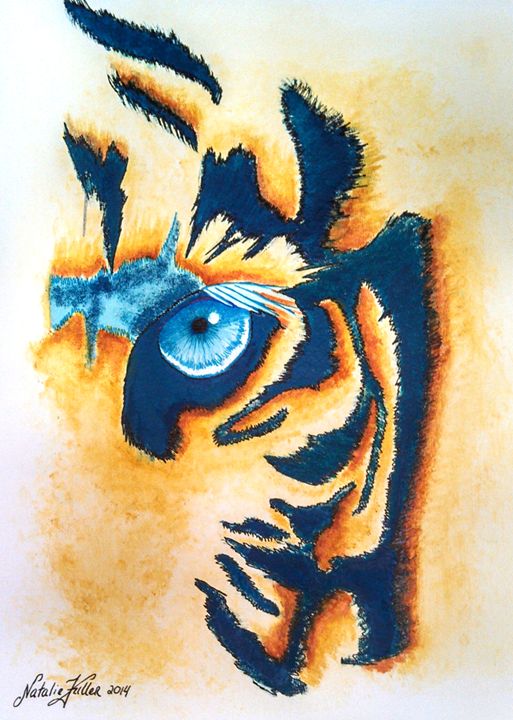This image is a detailed painting, likely watercolor, depicting the left half of a tiger's face. The artwork focuses intricately on the eye, which is a striking bright blue with a black pupil and a reflective white spot, resembling a human eye. Surrounding the eye, the tiger's fur is rendered with alternating patterns and colors - dark blue and black mixed with shades of orange and brown, though not in typical tiger stripes, giving it a unique abstract style. The fur around the eye features a hint of white and distinct lash-like lines. The lower left corner of the painting is signed in black script as "Natalie," with the ambiguous surname possibly being Fuller or similar, and dated 2014. This signature appears to be handwritten.